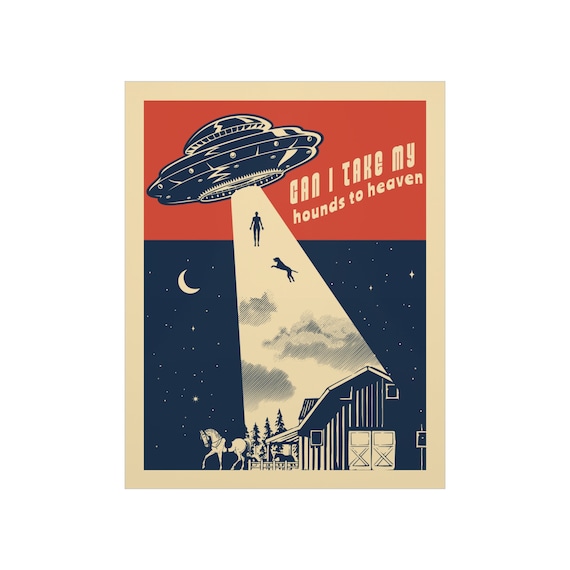This visually striking illustration is a three-color screen-printed poster with prominent beige off-white background resembling manila paper. Emphasized by its minimalist design and illustrative style, the poster depicts a night-time rural scene under a starry sky, including a navy blue crescent moon and various finely dotted stars. Central to the image, a blue UFO with white highlights hovers above, casting an orange-hued beam toward the ground. Within this beam, a person and a large dog, possibly a Mastiff, are being drawn up towards the UFO. Below, a serene countryside is portrayed with a white horse sporting a blue saddle and bridle standing in front of a barn. The barn is detailed with blue outlines and features white barn doors amidst a fenced yard and surrounding trees. A red stripe at the top of the poster distinctly frames the text "Can I take my hounds to heaven?" in white, adding a poignant or whimsical touch to the extraterrestrial scene.